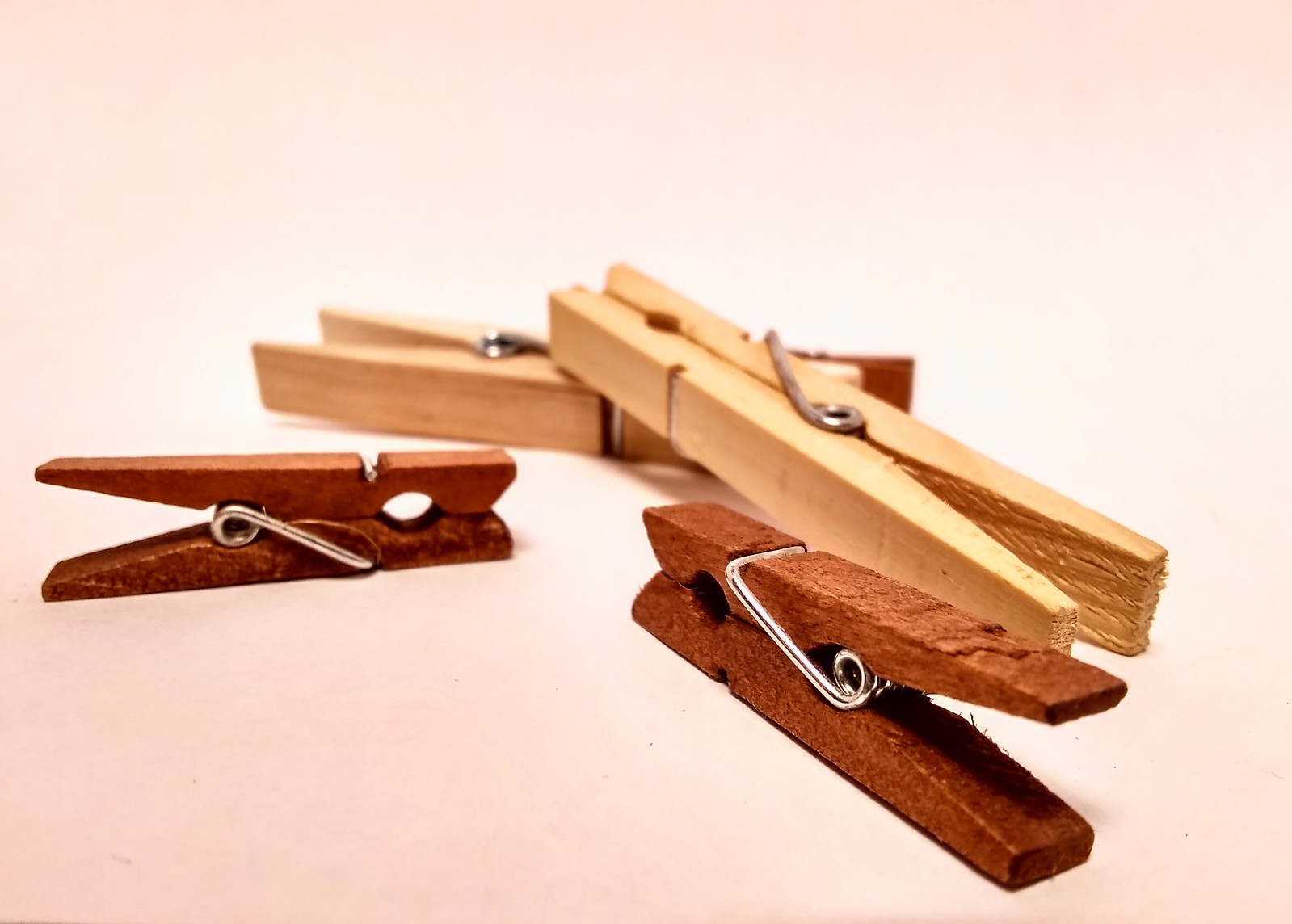This is an artistic close-up digital photo of four wooden old-style clothespins, showcasing a combination of darker and lighter wood tones against an extremely white background. The forefront clothespin, positioned on the bottom right, is a dark, rough-textured wood with a silver metal hinge spring facing downwards. Adjacent to it, on the left, another dark clothespin opens to the left, exhibiting the same wood and metal features. In the background, two larger clothespins of a nearly white, natural wood color intersect: one points diagonally towards the upper left while the other overlays it, angled towards the bottom right. The overall image suggests an intricate play of light and shadow, possibly enhanced to accentuate the contours and textures of the clothespins, creating a sense of depth and dimension on the otherwise stark white surface. The bottom left corner of the photo is slightly darker, adding a subtle contrast within the composition.